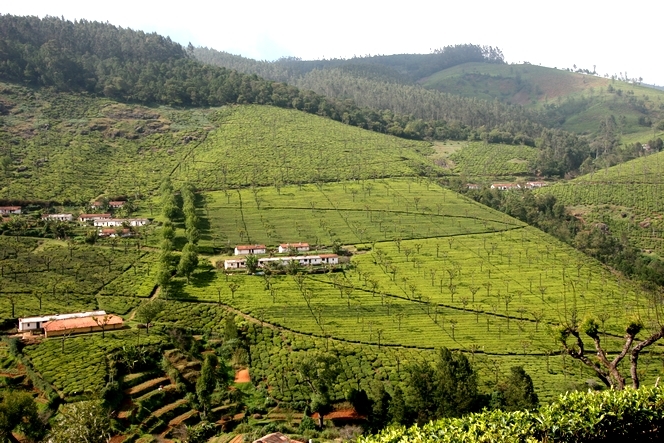The outdoor image captures a scenic, expansive green area viewed from a high vantage point, likely a hill or mountain top. The foreground showcases an array of green bushes to the bottom right, with earthy steps leading up towards several homes scattered throughout the landscape. The homes, characterized by Tan roofs and elongated structures, are mostly positioned on the left and center of the image. A pathway of brownish earth material steps can be seen towards the bottom left. Trees without leaves dot the scene, indicating a seasonal transition or dormancy. The background features a stunning panorama of rolling hills and mountains, with a mix of green fields and brown patches. The top of the mountains is adorned with trees, adding to the lush and varied texture. Despite a gray, overcast day creating a somber and subdued atmosphere, the picture is endowed with a tranquil beauty, rooted in its rich and diverse natural elements.